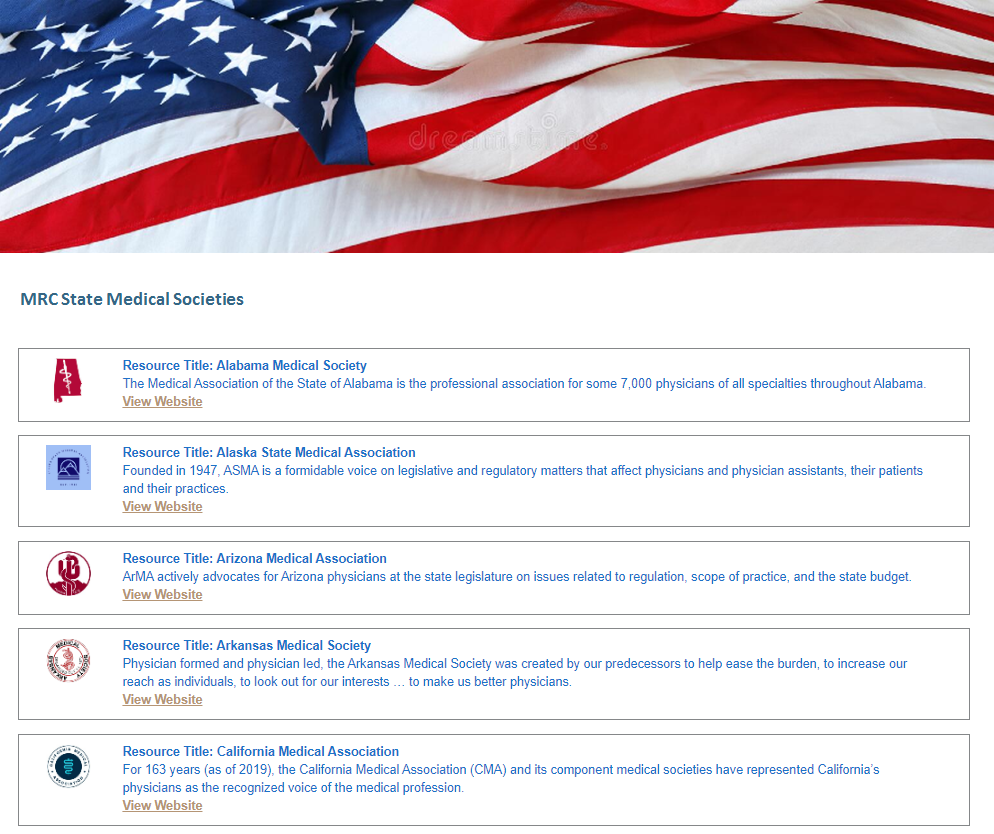Screenshot of a webpage displaying information about various state medical societies in the United States. 

At the very top of the page, there is a prominent American flag featuring the colors blue, red, and white, stretching from the left to the right. Just below the flag, the title "MRC State Medical Societies" is displayed in blue letters.

Directly underneath the title, there are five banner-like sections arranged horizontally across the page. Each banner contains details about a different state medical society:

1. **Alabama Medical Society**:
   - The banner includes an outline of the state of Alabama in red.
   - To the right of the outline, it says "Resource Title, Alabama Medical Society."
   - Descriptive Text: "The Medical Association of the State of Alabama is a professional association for some 7,000 physicians of all types of specialties throughout Alabama."

2. **Alaska State Medical Association**:
   - The banner features the title "Resource Title, Alaska State Medical Association."
   - Descriptive Text: "Founded in 1947, ASMA is a formidable voice in legislative and regulatory matters that affect physicians and physician assistants."

3. **Arizona Medical Association**:
   - The banner is labeled "Resource Title, Arizona Medical Association."
   - Descriptive Text: "ARMA actively advocates for Arizona physicians."

4. **Arkansas Medical Society**:
   - The banner bears the title "Resource Title, Arkansas Medical Society."

5. **California Medical Association**:
   - The banner features the title "Resource Title, California Medical Association."

Each section provides a quick insight into the primary role and formation of these medical societies, ranging from advocacy and professional support to their founding dates and the scope of their influence.